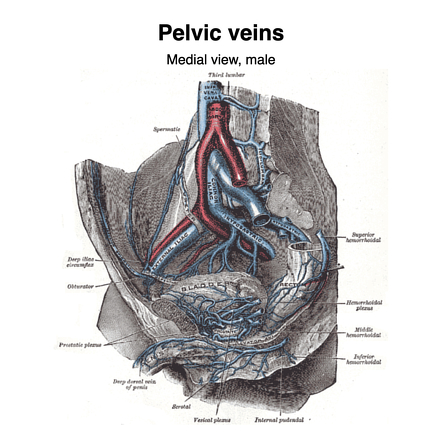The image is a detailed colored medical diagram depicting the pelvic veins from a medial view of a male. Set against a light, off-white background, the image is annotated with black text at the top that reads "Pelvic Veins" followed by "Medial View Male." Further down, in smaller, less legible text, it mentions "third something." The diagram itself presents the pelvic region in a grayish hue, highlighting internal structures with blue veins that branch out intricately alongside a prominent red artery. Annotations with lines point to various parts of the pelvic anatomy, although most of the text is too small to be readable, a few labels such as "bladder," "rectum," and "penis" are discernible. The bladder is depicted as an oval-shaped sac, while the rectum is shown as a hollow tube extending from it. The veins and arteries are color-coded for clarity, with blue representing the veins and red indicating the arteries. The rest of the image is shaded in a tannish color for better contrast among the labeled parts.